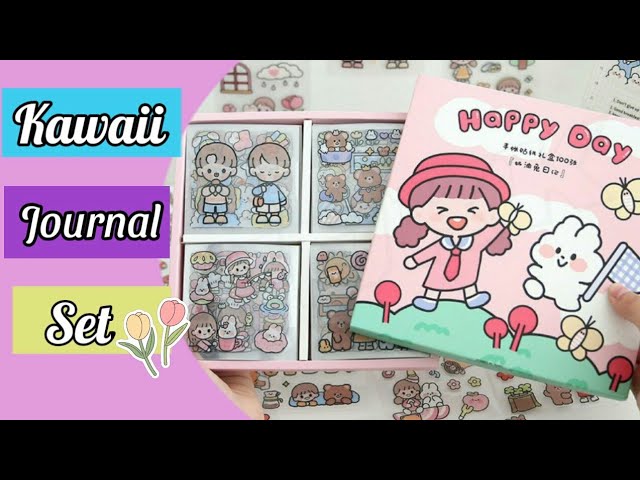This horizontally aligned rectangular image features a thick black border at the top and bottom, with vibrant graphic elements and text centrally aligned and framed on the left side. The text, organized vertically in white letters outlined in black, consists of three words on different colored backgrounds: "K-A-W-A-I-I" on a blue background, "journal" on a purple background, and "set" on a yellow background. Adjacent to the word "set," there are two charmingly drawn flowers—one yellow and one pink—each with leaves attached to their stems.

The right side of the image showcases the contents of the journal set, divided into four square sections. These sections display various animated characters: two charming characters in the first, a group of teddy bears in the second, a collection of characters in the third, and a card lying on top of these panels. The card, held by a visible hand from the right side, is adorned with the text "happy day," featuring an animated little girl with brown hair in a pink top and red tie, happily jaunting on green grass. The card’s background is pink, and it features three yellow bees, a cloud with eyes and a smile adorned with pink cheeks, and red mushrooms dotting the green landscape, adding to the whimsical, youthful aesthetic of the set.